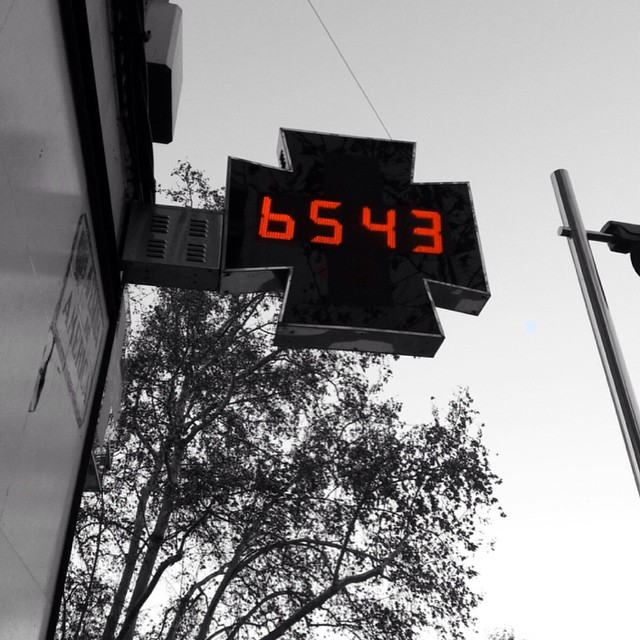A black and white photograph captures the quintessential essence of a European street scene. The image is taken from a low angle, showcasing a building facade prominently featuring a pharmacy sign. Unlike typical pharmacy signs that are usually green or bear the word "pharmacy," this one displays digital red numbers reading "6543." The pharmacy symbol, resembling a four-leaf clover with square edges, is attached just below a small ventilation grille with rows of slits.

To the left, partially visible on the building wall, is a street sign starting with the letter "A," possibly indicating the name "Amari" or "Amarik," presented on small tiles, a common European style. On the right, a street pole is visible, standing sentry next to a large, sprawling tree whose branches and leaves are intricately detailed against the backdrop of the sky. Overhead, a network of electrical or telephone lines crisscrosses the scene, adding to the urban ambiance. The sky appears dreary and overcast, suggesting possibly foggy weather, even in the monochrome palette of the photograph.